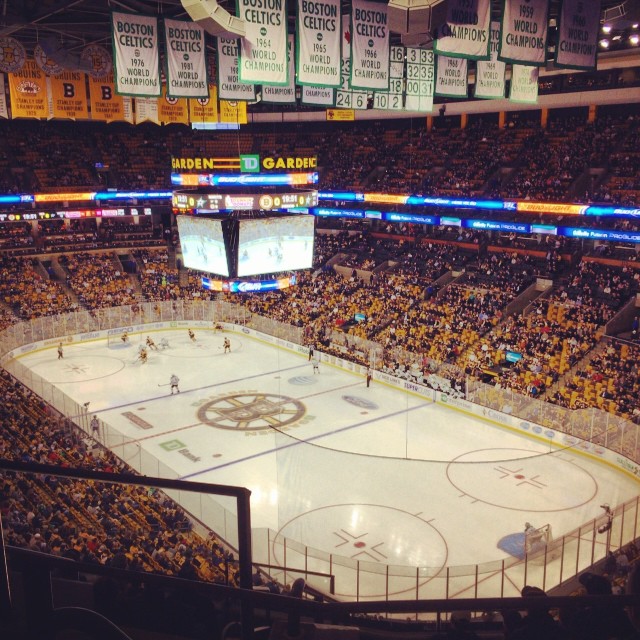This image captures an aerial view of a Boston Bruins hockey game at the TD Garden, taken from a high vantage point, likely from a balcony or upper stands. The center of the image features the ice rink with the distinctive spoked 'B' Boston Bruins logo at center ice. Hockey players and referees are scattered across the ice, with one lone goalie positioned near the bottom of the picture.

Surrounding the rink are stands filled with spectators mainly dressed in black and yellow, seated in predominantly yellow seats. The stands, also visible on the left, right, and extending to the top of the image, have a few empty sections but are mostly packed with fans. The upper facade of the arena has blue borders that encircle the stadium.

At the very top of the image, various banners hang from the rafters. These include white and green Boston Celtics banners, as well as yellow and black Boston Bruins banners. Centered but slightly to the left below these banners hangs the jumbotron, which prominently displays "TD Garden" and features multiple screens showing the game's action from different angles. The jumbotron incorporates blue, black, yellow, and green colors.

The overall scene conveys the energy and excitement of a professional hockey match, set in the iconic Boston Garden arena.